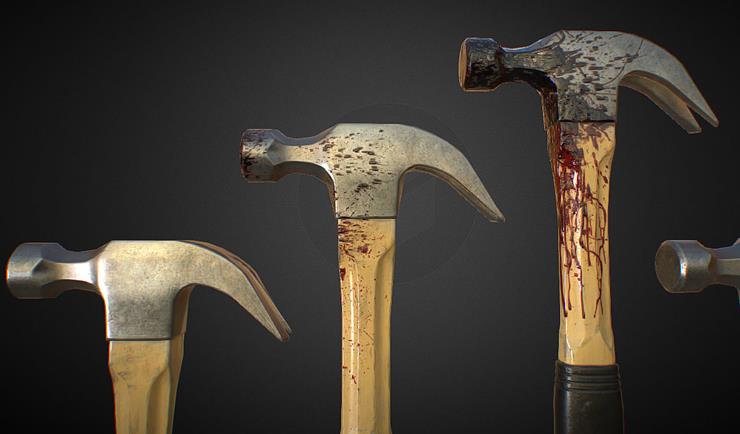In the image, four hammers are displayed against a blackish-gray gradient background, arranged in a diagonal pattern ascending from the lower left to the upper right, then descending slightly. Each hammer has a dull yellow wooden handle with a silver metal head. The hammer on the far left has a clean, shiny head and handle. The second hammer, positioned slightly higher, shows a small amount of red substance, resembling blood, splattered on its head and side. The third hammer, which stands the tallest and has a black rubber grip section beneath the dull yellow wood, is heavily covered in the red substance, with splatters on the tip, head, and dripping down the handle. The fourth hammer, slightly lower than the third but to its right, shows only the clean tip of the head. The entire image is contained within a long vertical rectangle, emphasizing the gradual change in the condition of the hammers from clean on the left to blood-splattered on the right.